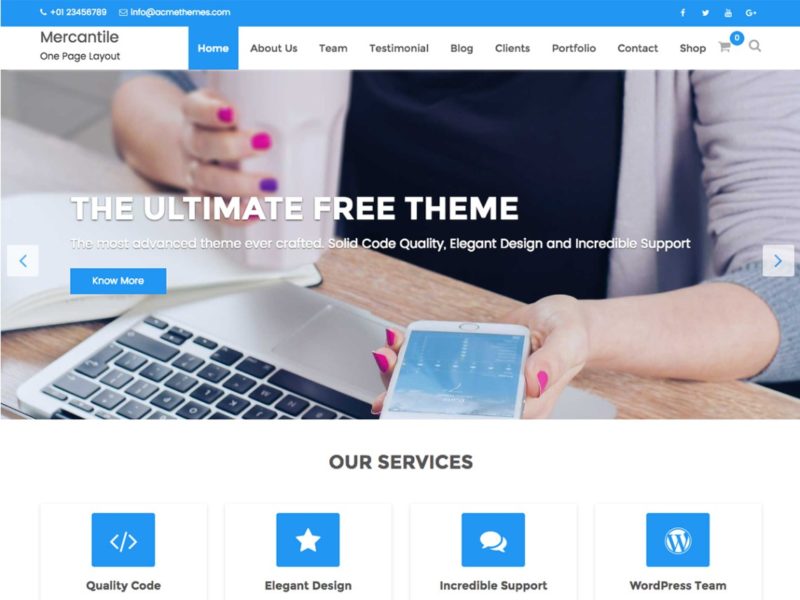The top left corner of the image features the text: "Plus, Zero, One, Two, Three, Four, Five, Six, Seven, Eight, Nine," followed by "Help" and "Info at acmethermies.com." Social media icons for Facebook, Twitter, YouTube, and Google+ are displayed. The navigation menu includes options for "Right Control," "One Page Layout," "Home," "Virus," "Team," "Testimony," "Blog," "Plan," "Portfolio," "Contact," "Shop," and a "Shopping Cart" with zero items. 

In the center of the image is a person with a colorful nose, accompanied by the text "This is the ultimate free theme." The person holds a phone in their hand, which displays a weather update of 7 degrees. The image also shows a wooden table.

Beneath, there's a section titled "Our Services," displaying four pictures labeled "Quality Code," "Elegant Design," "Incredible Support," and "WordPress Team." Navigation arrows are situated on either side of this section, with additional symbols like a slash and a star in blue. Various speech bubbles containing texts are scattered around, reinforcing the focus on the WordPress team.